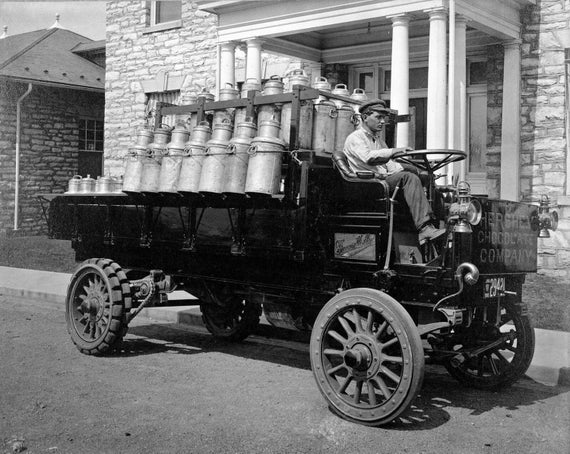This antique black-and-white photograph captures a very old delivery truck from Hershey's Chocolate Company. The truck is simple, mechanical, and blocky in design, with rigid and hard-looking wheels, and it is entirely open without a cab. The driver, a man wearing a gray cap and a white shirt, is seated in open air, steering the vehicle with a large wheel and basic controls. The front of the truck prominently displays the name "Hershey's Chocolate Company" within a black rectangle. Behind the driver, the truck is loaded with numerous cylindrical, metal barrels that resemble milk jugs, arranged in a pyramid-like stack. Additionally, there is a wooden crate holding even more of these pressurized-looking cylinders. The truck appears to be parked on a gravel road in front of a brick building with four columns at the door. The setting and vehicle evoke a bygone era, highlighting the early days of industrial chocolate delivery.